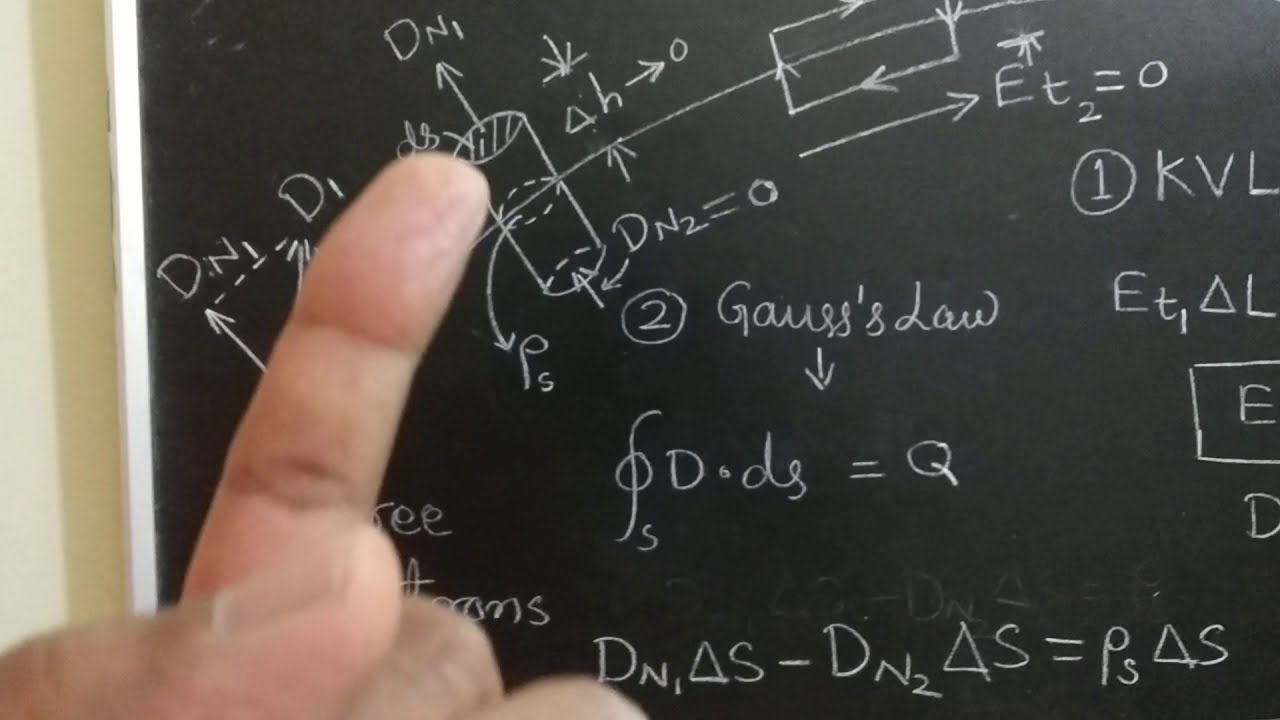In this close-up image, the primary focus is a blackboard densely covered with complex mathematical formulas and diagrams. The background is an off-white color, creating a stark contrast with the blackboard that spans most of the frame. Prominently, the index finger of a man's hand, located in the bottom left corner, points toward a section of the chalkboard. This hand also partially reveals the thumb and other fingers.

The chalkboard itself is crowded with various equations and illustrative diagrams drawn in white chalk. Notably, in the upper left quadrant, there is a cylindrical shape labeled "DN1," suggesting it might relate to a formula involving cylindrical objects or electrical currents. Numerous arrows and additional notations, such as “Gauss's Law” and “DN1 triangle S minus DN2 triangle S equals PS triangle S,” are visible, indicating a highly technical and mathematical context. The overall setting appears to be indoors, possibly in a classroom or lecture hall, though the specific time of day is indiscernible.